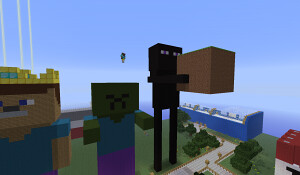In this detailed scene from a game resembling Roblox, a group of distinct characters are assembled at the edge of a lofty area, seemingly high above a landscape dotted with blocky, tree-like structures. The first character stands out with a bright yellow crown, exuding a regal air. Next to them is a quirky figure with a green head and a blue shirt, adding a splash of vibrant color to the group. Towering above these two is a mysterious and imposing character, cloaked entirely in black with striking purple eyes, gripping a brown box with an air of importance. The environment around them is a fascinating blend of digital and Lego-like aesthetics, characterized by large, blocky constructions. A prominent blue structure looms behind the group, its significant size suggesting it is an important feature of the scene. Red blocks are scattered nearby, adding more color to the setting. The entire ensemble is perched in an outdoor, high-altitude environment, creating a sense of adventure and exploration.